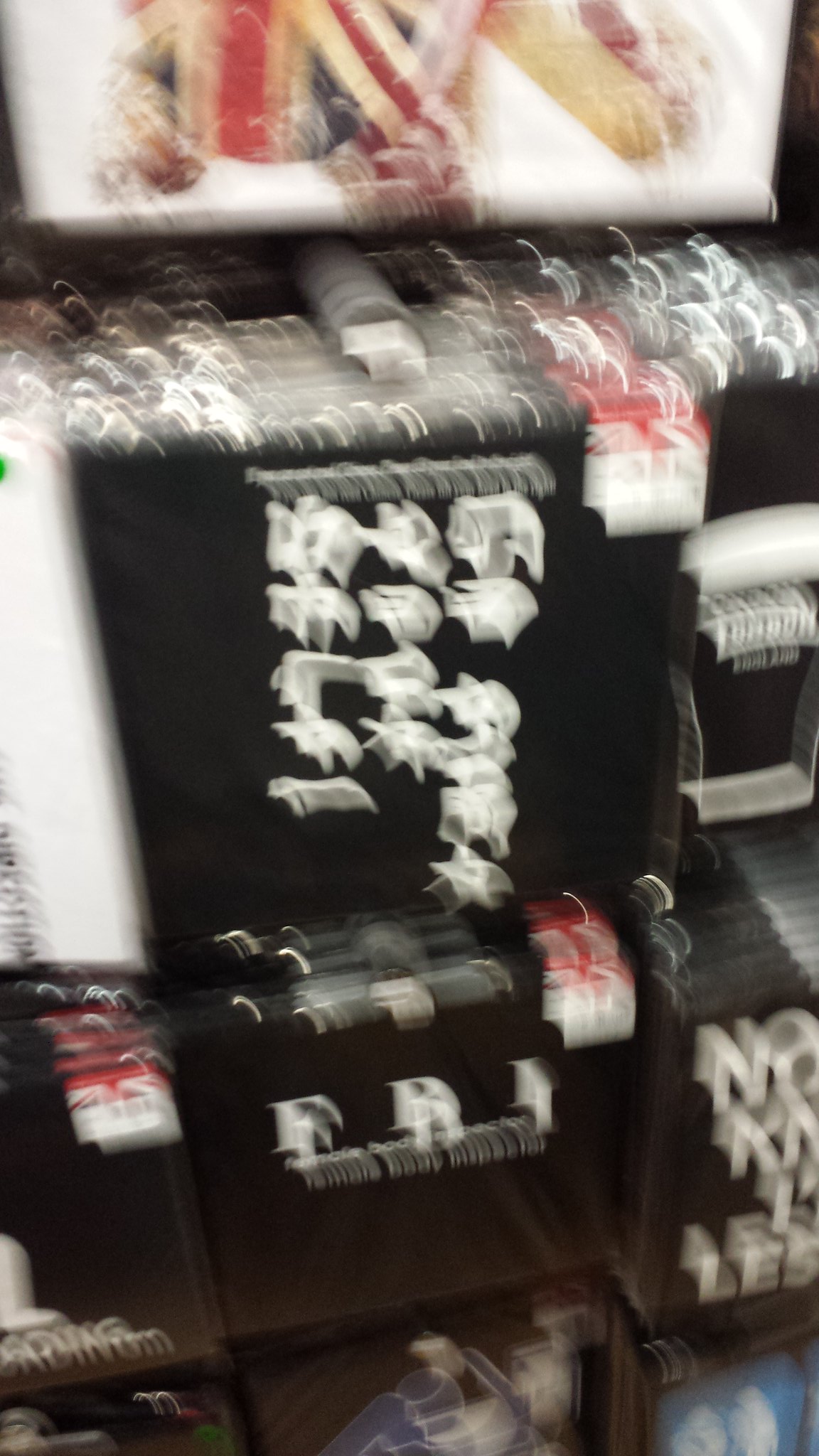The image appears to be taken in a store setting, showcasing several black square packages or placemats with distinct white and red tags located on the top right corner. The upper section of the tags is red with white text, while the lower section is white with black text. The packaging features white figures, some resembling animals or birds. These items are hung on white plastic hangers with gray ends, and at least eight of these packages are visible, arranged across multiple racks. Above these racks, there's a white sign adorned with yellow, red, and black elements, along with a prominent red and white 'M'. The overall scene is slightly blurred, but suggests a well-organized retail display.